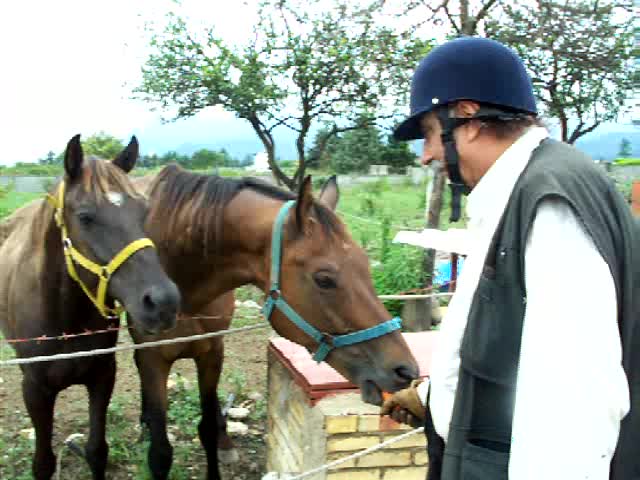In this detailed photograph, an elderly man with a gray mustache, wearing a dark blue helmet with a black chin strap, is feeding a carrot to one of the two horses in front of him. Both horses have straight brown fur and a black mane, with light brown tips at the end. Their large, black eyes are accentuated by their perked ears, which are darker at the edges and lighter on the inside. The horse on the left sports a very dark brown or almost black face, contrasted by the horse on the right, which has a more brown face with a black mouth, and a blue strap around its head and face. The horse on the left, which is awaiting its turn, has a yellow strap around its face and head.

The serene backdrop features a bright blue and white sky, a green field, and several skinny trees crowned with lush green leaves. A white fence topped with barbed wire runs behind the horses, adding to the rustic charm. The man, attired in a black vest over a long-sleeved white jacket and brown gloves, grins as he holds an orange carrot up to the mouth of the horse on the right. The clarity of the image is slightly compromised, indicative of a lower-quality camera, but the scene is warm and captures a tender moment likely meant for personal reflection.